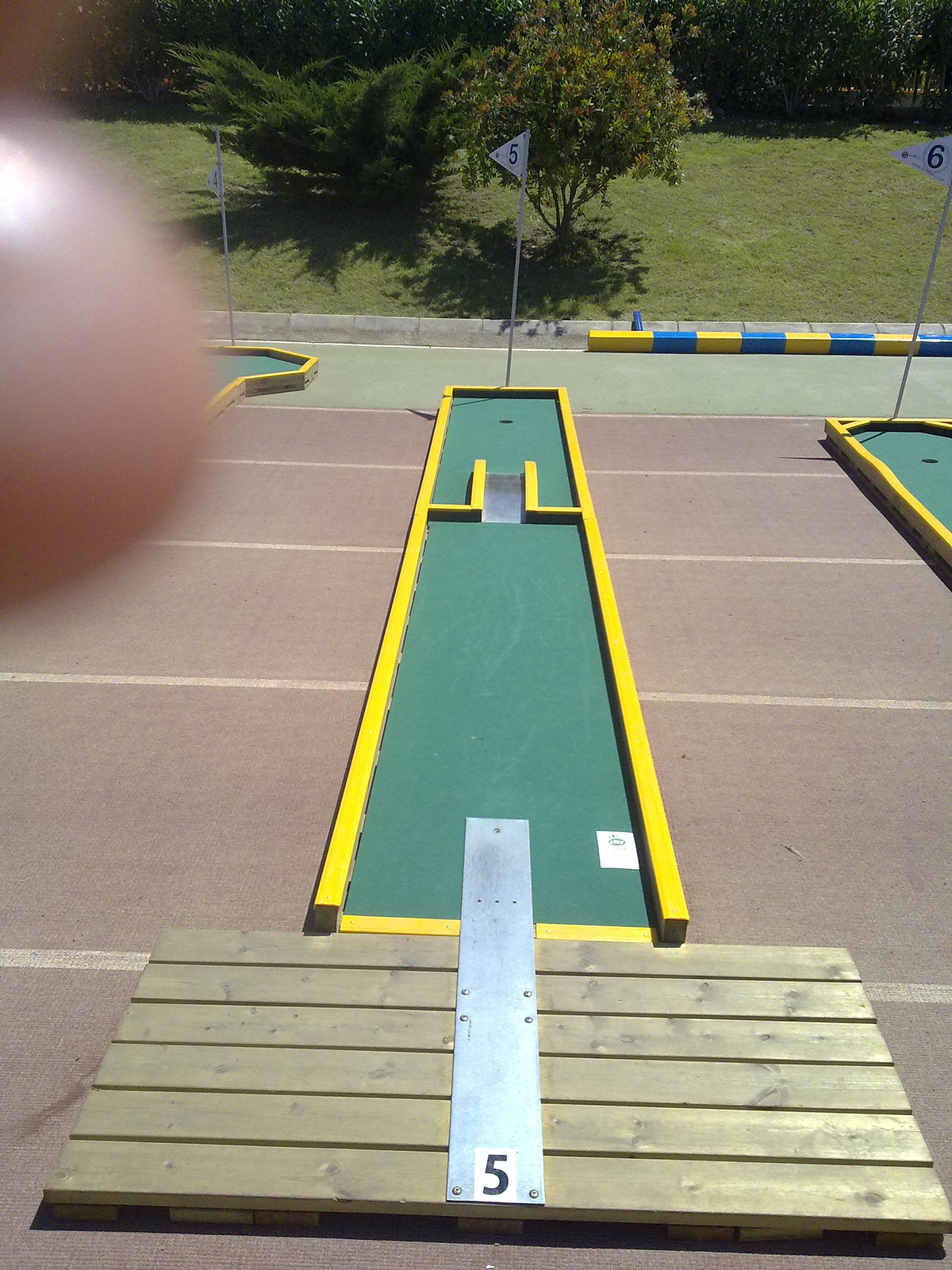The image depicts the fifth hole of a mini golf course set in a park-like area. In front of the frame, there is a structure made up of six wooden planks with a metal strip running across them, which holds a white rectangular sign marked with the number "5." This indicates the start of the hole. The course itself is a 40-foot long rectangular green fairway bordered by yellow barriers. Near the middle of the fairway, two yellow boards create a narrow passage that players must putt through. Just beyond this narrow section lies the hole, marked by a flag labeled with the number "5."

In the background, one can see parts of the neighboring holes, with the fourth hole partially visible to the left, obscured slightly by the photographer’s finger, and the sixth hole cut off by the right edge of the image. The area is bordered by a concrete culvert and a wooden barrier painted in alternating colors of white, yellow, and blue in one-foot strips. At the top edge of the course, there's a walking path separating the mini golf area from a field with grass, bushes, and trees, allowing visitors to walk without stepping on the course itself. The field also features a brown pavement with white lines running every 20 feet horizontally.